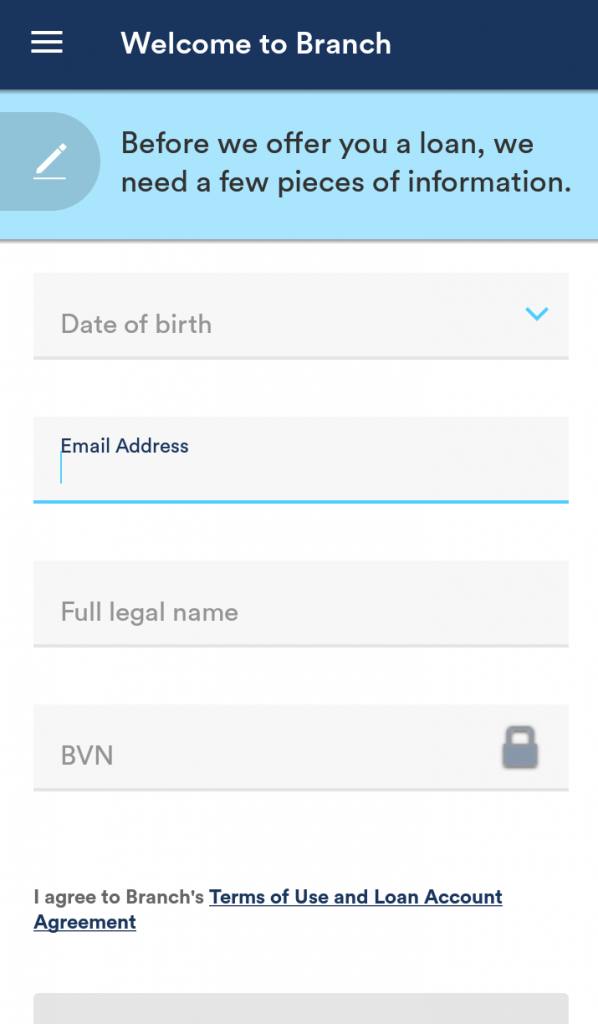Screenshot from the "Welcome to Branch" app during the installation stage. The app, having just been installed, is prompting the user to provide additional information required for offering loan products. The user interface requests the date of birth, email address (currently being filled in by the user), full legal name, and BVN (Bank Verification Number). At the bottom, there is a hyperlink to the app's terms and conditions, which are mandatory for proceeding with the loan application. There are three white lines at the top adjacent to the "Welcome to Branch" title, indicating a menu for accessing more options and information before submitting the loan request.